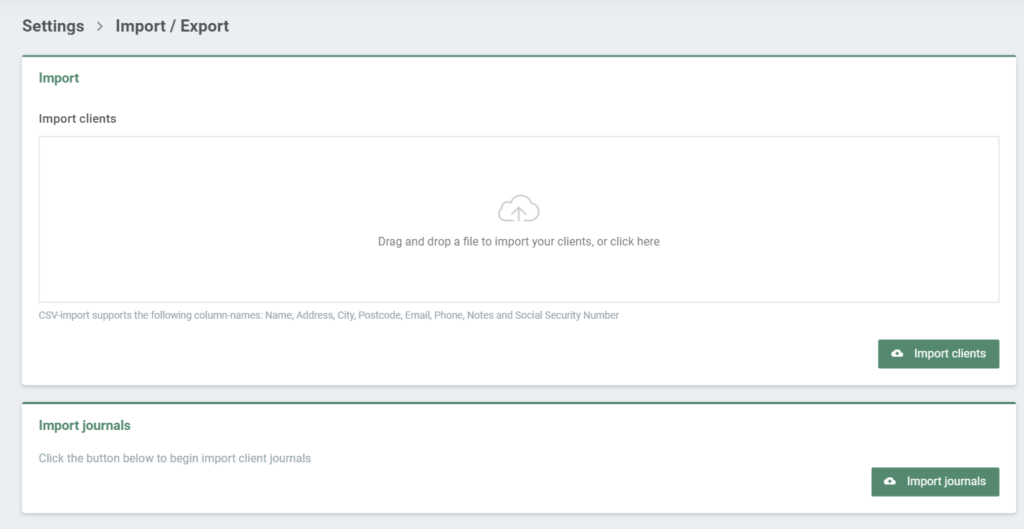This is a detailed screenshot of a computer screen, featuring a user interface for import/export settings. The background is a very light blue, almost grayish hue. In the upper left corner, the black font text reads "Settings > Import/Export".

Below this are two white boxes, one beneath the other, with the first box being larger. 

**First White Box:**
- Upper left corner features the label "Import" in green.
- Below this, in a standard font, is the text "Import Clients".
- Inside a light gray sub-box within the larger box, you see a cloud icon with an upward arrow above a prompt that reads "Drag and drop a file here to import your clients or click here".
- Small fine print on the left side of the white box states "CBS import supports the following" with additional unreadable text.
- Lower right corner houses a green "Import Clients" button.

**Second White Box:**
- Upper left corner is marked with the label "Import Journals".
- Below it, the instructions read "Click the button below to begin importing client journals".
- The box also contains a thin green border at the top.
- Lower right corner features a green "Import Journals" button.

Overall, the screenshot captures a straightforward, easy-to-navigate interface for importing clients and journals, marked by clear labels and intuitive user prompts.